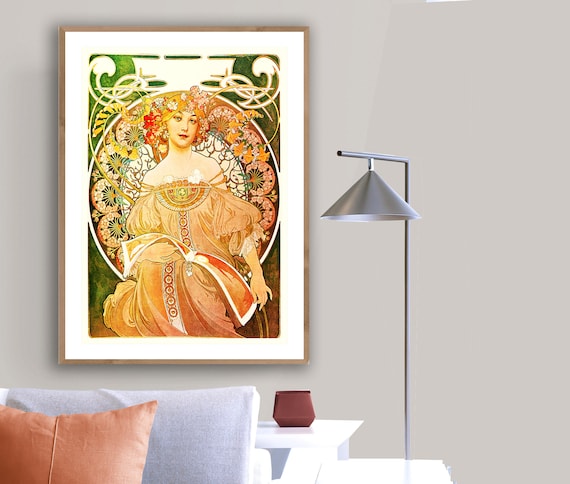The image depicts a serene section of a living room featuring a light gray wall that serves as a backdrop to a beautifully arranged setting. Centered in the scene is a gray sofa with a bit of tan hues, complemented by an orange pillow that adds a pop of color. Beside the sofa stands a sleek, metallic lamp with a thin pole and a lampshade directed towards the floor, casting a cozy light over the area.

Dominating the upper portion of the wall is a large framed artwork. The art piece showcases a classical woman reminiscent of the Victorian era or a goddess figure. She is adorned in a peach or orangish-red dress with poofy sleeves and sits gracefully on a chair with floral details. Her hair is decorated with flowers, and she holds an open book, gesturing with one hand towards the text while the other points downward. The artwork is encapsulated in a thick white-bordered frame, adding a genteel touch to the overall aesthetic. This thoughtful composition of colors, textures, and art creates a harmonious and inviting living space.